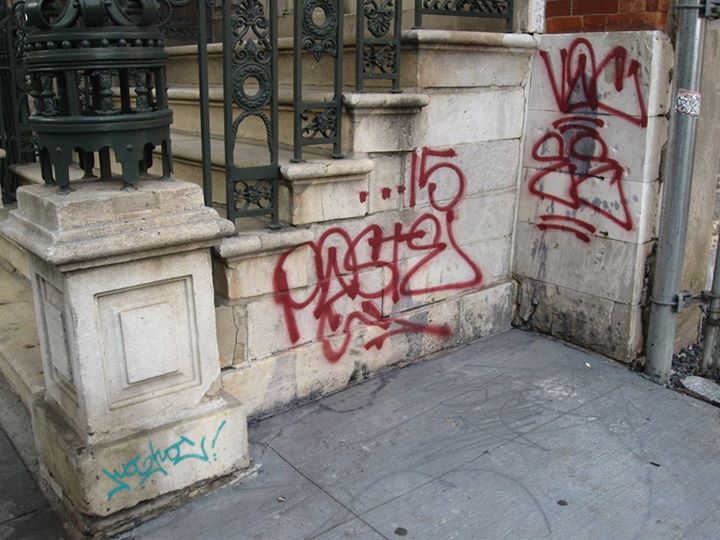The photograph captures a section of a city sidewalk featuring a notable set of stone steps leading up to a stoop. These steps, made of white stone, are flanked by a black wrought iron railing. Adjacent to the steps, there is a small, three-foot-high metal pillar topped with intricate ironwork. The ground is composed of large, gray, rectangular tiles, giving the sidewalk a solid, urban feel. A brick wall beside the stairs prominently displays graffiti; on its lower section, blue spray-painted graffiti catches the eye near the metal pillar, while higher up, red graffiti sprawls across the wall and the side of the steps. This graffiti includes the artist's tag "pasty," a scribbled marking, the number 15, and a small sketch resembling a crown followed by two eyes and several triangles. The scene is a detailed snapshot of urban life, capturing both the built environment and the spontaneous art that adorns it.